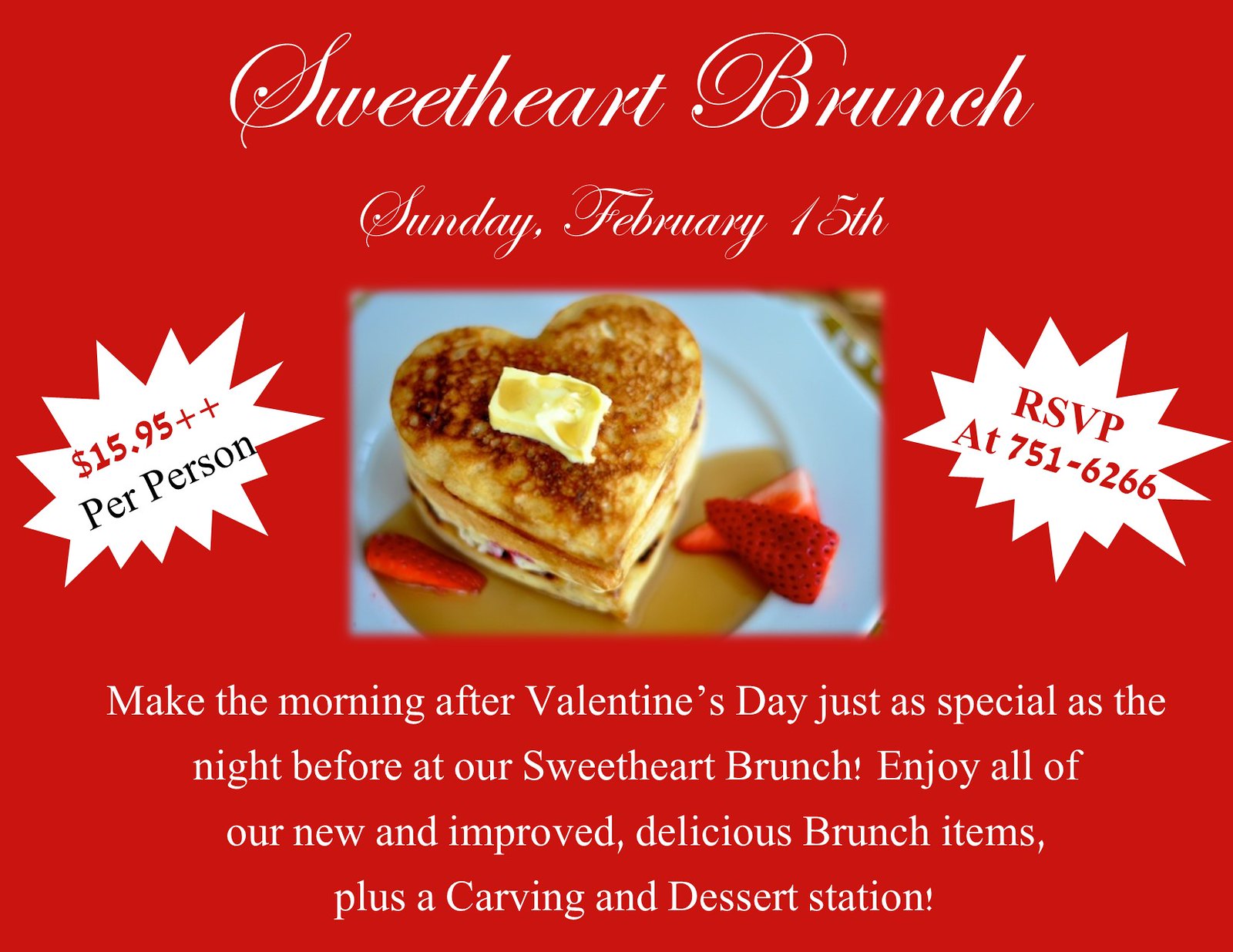The advertisement features a vibrant red background with elegant white cursive text at the top that reads "Sweetheart Brunch." Directly beneath, it announces “Sunday, February 15th.” Central to the ad is a visually appealing photo of heart-shaped pancakes on a blue plate, garnished with a few fresh strawberries and drizzled with syrup. On the left side, within a white starburst design, is the pricing detail "15.95++" in red font, with "per person" in black font. Mirroring this on the right side, another white starburst contains the RSVP detail "RSVP at 7516266" in red font. At the bottom of the ad, a compelling tagline in white font invites patrons to "Make the morning after Valentine's Day just as special as the night before at our Sweetheart Brunch. Enjoy all of our new and improved delicious brunch items plus a carving and dessert station!"